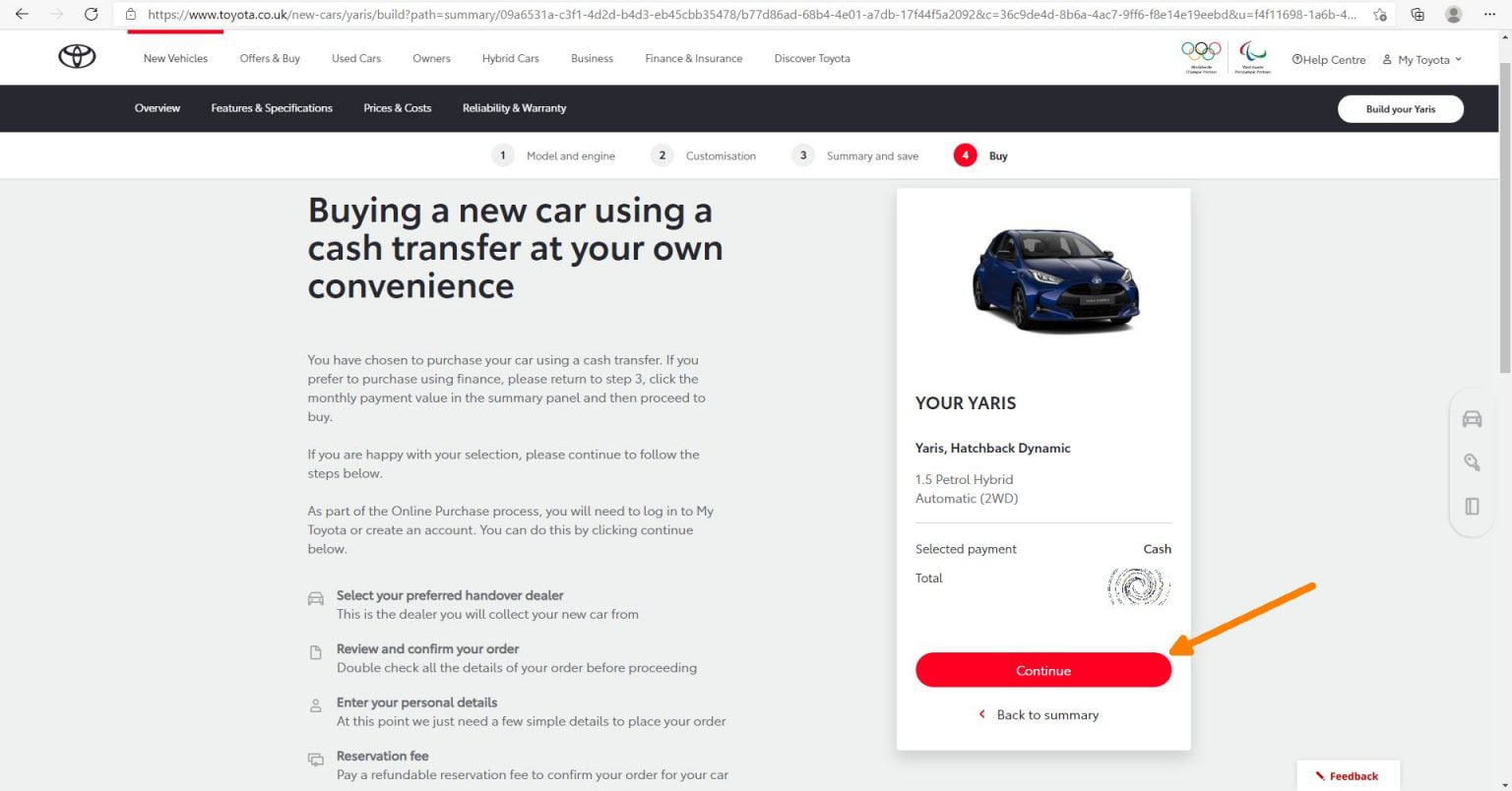This detailed caption describes the image from a web page displayed on a smart device or computer screen:

The image is a left-to-right horizontal screenshot of a Toyota web page. At the top left, there is a backward-pointing arrow, and beside it, a grayed-out forward arrow indicating no forward navigation is currently available. Next to these is a refresh button. To the right of these navigational elements is a white web address bar, underlined in red at the start. Further to the right, there are various icons including a user profile icon, and three horizontal dots representing more options.

On the left side of the page, there is a Toyota car emblem. Below this logo are several navigation options, such as "New Vehicles," "Offers & Buy," "Used Cars," "Owners," "Hybrid Cars," "Business," "Finance & Insurance," and "Discover Toyota." An Olympic symbol is also present to the right of these navigation links, followed by a help center symbol, and the "myToyota" account app icon.

A black strip runs horizontally below these elements, with white text listing sections like "Overview," "Features and Specifications," "Prices and Costs," and "Reliability and Warranty." Underneath this strip, the webpage outlines a four-step process for buying a car which includes: 1) Model and Engine, 2) Customization, 3) Summary and Save, and 4) Buy. The fourth step is emphasized in red, while the others are gray. The buy step includes details about purchasing a new car via cash transfer at the user's convenience.

Further down, a picture of a Yaris model is displayed alongside information about the vehicle. Buttons labeled "Continue" and "Back to Summary" are available for navigation. In the bottom right corner of the page is a button for providing feedback.